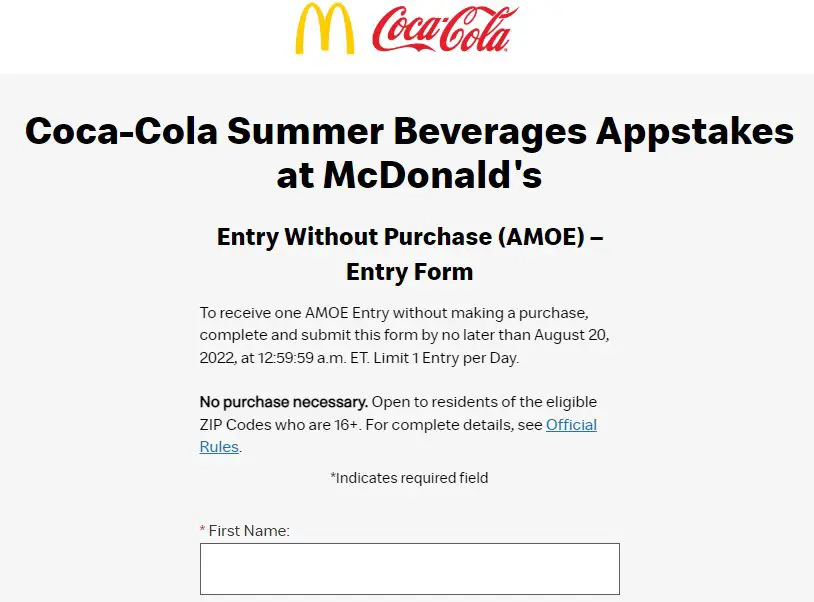The top of the image prominently features a yellow McDonald's logo ("M") alongside a red Coca-Cola logo, all set against a white background. Below these logos, there is a gray box containing text that promotes the "Coca-Cola Summer Beverage Sweepstakes at McDonald's." The text reads: "Enter without purchase (AMOE) – Entry Form."

To participate without making a purchase, individuals are instructed to complete and submit the form by August 20, 2022, at 12:59:59 a.m. Eastern Time. The caption specifies a limit of one entry per day and emphasizes that no purchase is necessary. The promotion is open to residents of eligible zip codes who are 18 years or older. For full details, participants are directed to see the "Official Rules," with "Official Rules" being highlighted in blue, while the rest of the text is in black.

An asterisk indicates that certain fields are required, such as "First Name," next to which there is an asterisk. There is a corresponding white data field edged in dark gray for entering the first name, indicating that more information fields likely follow beyond the showcased section. The color scheme of the image includes yellow, red, black, gray, blue, and white, reflecting the branding of both McDonald's and Coca-Cola. Text within the gray box references the Coca-Cola Summer Beverage Sweepstakes at McDonald's and details how to enter without a purchase (AMOE) through the provided entry form.